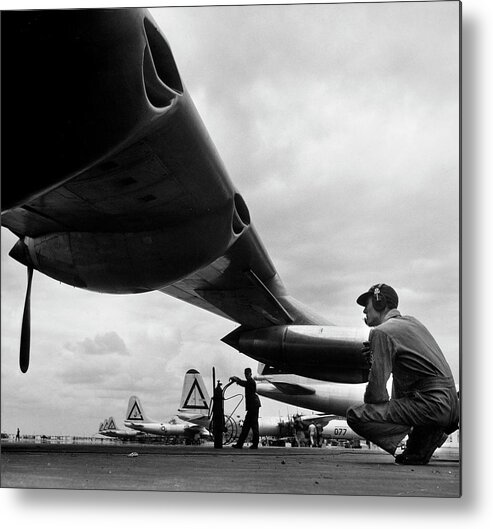The black-and-white photograph captures a bustling airfield, reminiscent of a bygone era. Dominating the foreground, a large airplane wing extends diagonally from the upper left corner to the middle of the frame. Beneath this wing, a man in a flight suit crouches on the pavement, wearing a black baseball cap and soundproof earmuffs. His attention is fixed on the aircraft's engine, suggesting he might be conducting an inspection or maintenance.

Further back, more aircraft populate the scene. These planes, distinguished by their prominent black triangle logos on the tails, appear to be military or private jets. The sky above is filled with a mix of gray and white clouds, casting a somber tone over the image.

Additional figures are scattered across the airfield. One man, positioned near the wing, holds a piece of equipment that could be an oxygen tank or another tool vital for aircraft servicing. Other individuals are visible between the tail fins of the distant planes, likely engaged in conversation or further technical tasks.

This meticulously composed photograph, through its grayscale palette and detailed elements, offers a nostalgic glimpse into aviation history, highlighting both the human and mechanical aspects of early air travel.